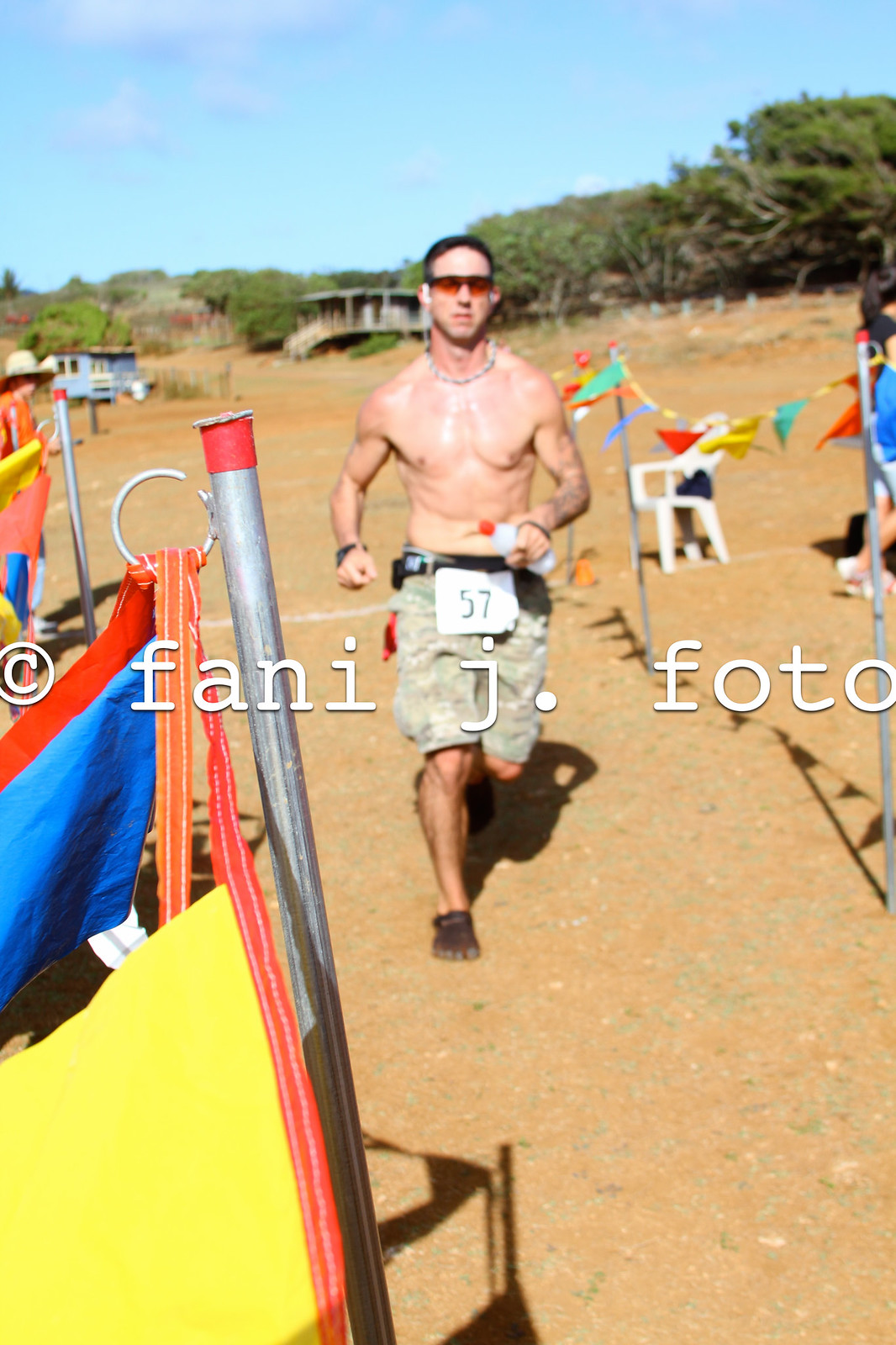In this detailed image, a shirtless, muscular man is seen running, likely participating in a marathon or similar event. He is clad in greyish cargo shorts bearing number 57 on a white paper attached to his waist. He accessorizes with dark sunglasses, short dark hair, a necklace, and earpods, and he has tattoos down his left arm. In one hand, he carries a water bottle with a red cap, while a red shirt hangs from his back pocket. The man is wearing brown sneakers and appears to be nearing the finish line.

The setting is a sandy beach, with a grey pole featuring a round strap and yellow and blue tarps to the left. A person in an orange top and light grey hat stands at the far left. Green trees and a grey hut with brown stairs adorn the background. A festive banner with blue, red, yellow, and lime green triangle flags drapes across the lower right. The course is marked with colorful flags and lined with some plastic chairs, and spectators can be seen, including one with a big sun hat. The scene is stamped with the watermark "FANI J PHOTO," adding a professional touch to the image.